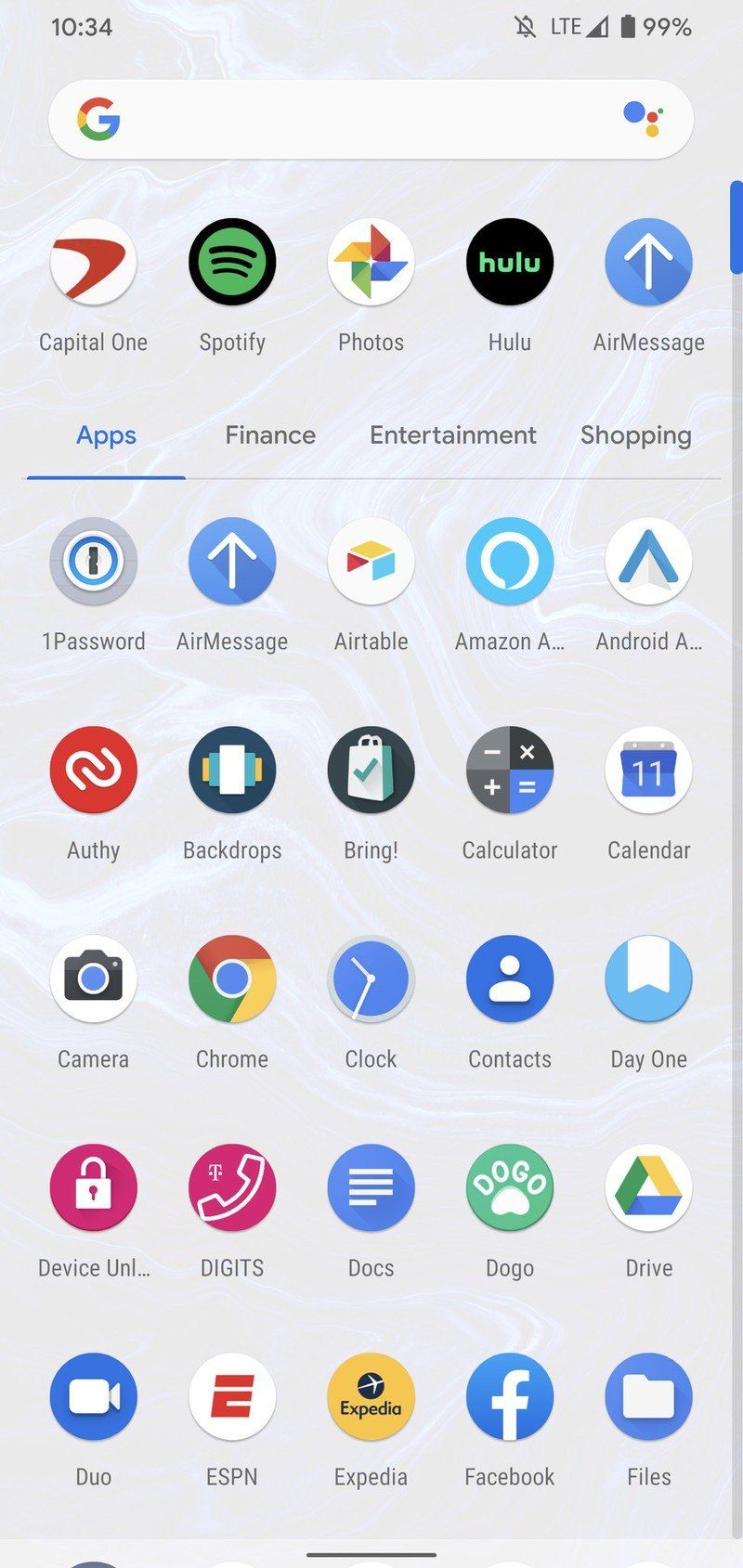This image captures the user interface of a smartphone displaying its home screen. The status bar at the top right shows a fully charged battery at 99%, LTE signal strength, and a muted ringer icon. It's 10:34 AM, as indicated by the digital clock.

Front and center is a Google search bar distinguished by its multi-colored 'G' logo, bordered by round icons on either side. Below this search bar, five prominent app icons are visible: Capital One, Spotify, Photos, Hulu, and AirMessage, the latter featuring a blue arrow pointing upward. 

Further down, a section title "Apps" is highlighted with a blue underline, segmented into categories such as Finance, Entertainment, and Shopping. Below these categories is a comprehensive list of app icons: 1Password, AirMessage, Airtable, Amazon, Android, Arthi, Backdrops, Bring, Calculator, Calendar, Camera, Chrome, Clock, Contacts, Day One, Device, UNI, Digits, Docs, Dogo, Drive, Duo, ESPN, Expedia, Facebook, and Files. 

There appears to be additional content below the visible area, as suggested by a small black image on the left side, indicating possible items cut off from the current view.